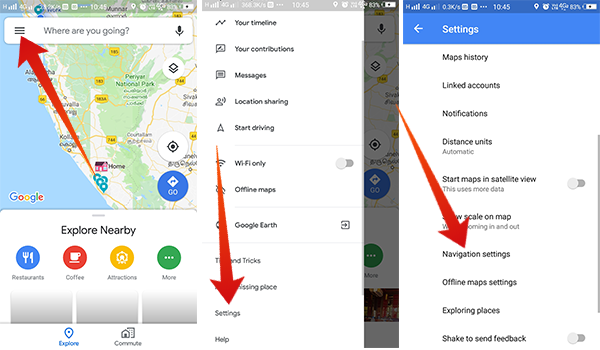The image features three smartphone screens laid out horizontally side by side, each showcasing different app interfaces and functions.

**Far Left Screen:**
- A text box at the top reads "Where are you going?" with a large red arrow pointing towards it, emphasizing its importance.
- Below the text box, there is a blurred map with a cluster of blue pins concentrated in one area.
- An image of a pink house labeled "Home" is also visible.
- At the bottom, icons for different categories such as "Restaurants," "Coffee," "Attractions," and more are displayed.

**Middle Screen:**
- This screen showcases a vertical column of various icons, each accompanied by descriptive text:
  - "Your Timeline"
  - "Your Contributions"
  - "Messages"
  - "Location Sharing"
  - "Start Driving"
  - "WiFi Only" (this option is currently disabled)
  - "Offline Maps"
  - "Global Earth"
- A large red arrow points downwards towards the "Settings" option.

**Far Right Screen:**
- The top of the screen displays "Settings" with multiple options listed below:
  - "Maps History"
  - "Linked Accounts"
  - "Notifications"
  - "Distance Units"
  - "Start Maps"
  - "Satellite View" (this option is disabled)
  - "Show Scale on Map"
- A large red arrow highlights the "Navigation Settings" entry.
- Additional options include "Offline Map Settings," "Exploring Places," and "Shake to Send Feedback."